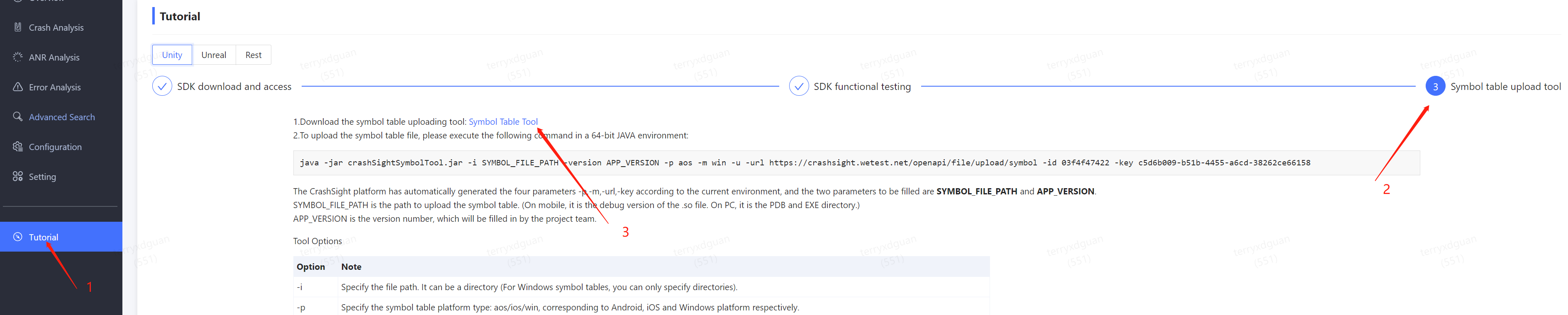### Caption for SDK Functional Testing Tutorial Image

This image illustrates an SDK functional testing tutorial screen. On the left side, a navigation pane lists several links: Crash Analysis, ANR Analysis, Error Analysis, Advanced Search, Configurations, Settings, and at the bottom, a link to Tutorial. The current focus is on the Tutorial tab.

On the right side, the heading "Tutorial" is displayed prominently, followed by three options: Unity, Unreal, and REST, indicating different frameworks or services. The current screen title is "SDK Downloading Access."

The tutorial instructs the following steps:
1. **Download the Symbol Table Uploading Tool**: The phrase "Symbol table tool" is highlighted in blue, indicating it is a clickable or downloadable link. A red arrow points to this link with the number "3" beneath it.

2. **Upload the Symbol Table File**: Users are prompted to execute a command in a 64-bit Java environment. The text explains that the Crash Site platform has automatically generated four parameters: `p`, `m`, `url-key`, in accordance with the current environment. Users need to fill in two parameters: `symbol_file_path` and `app_version`.

   - `symbol_file_path`: Path to the symbol table, denoted in different formats based on the platform (e.g., on mobile it refers to the debug version of a .so file; on PC, it refers to the PDB and EXE directory).
   - `app_version`: The project team will fill this in with the version number.

Below this section, two options are specified:
- **Option I**: This option notes the need to specify the file path, which can be a directory for Windows symbol tables, limited to directories only.
- **Option P**: This option requires specifying the symbol table platform type, using codes AOS/iOS/win corresponding to Android, iOS, and Windows platforms respectively.

The detailed structure and step-by-step instructions highlight the practical aspects of using the SDK Downloading Access page, providing a comprehensive guide for users.